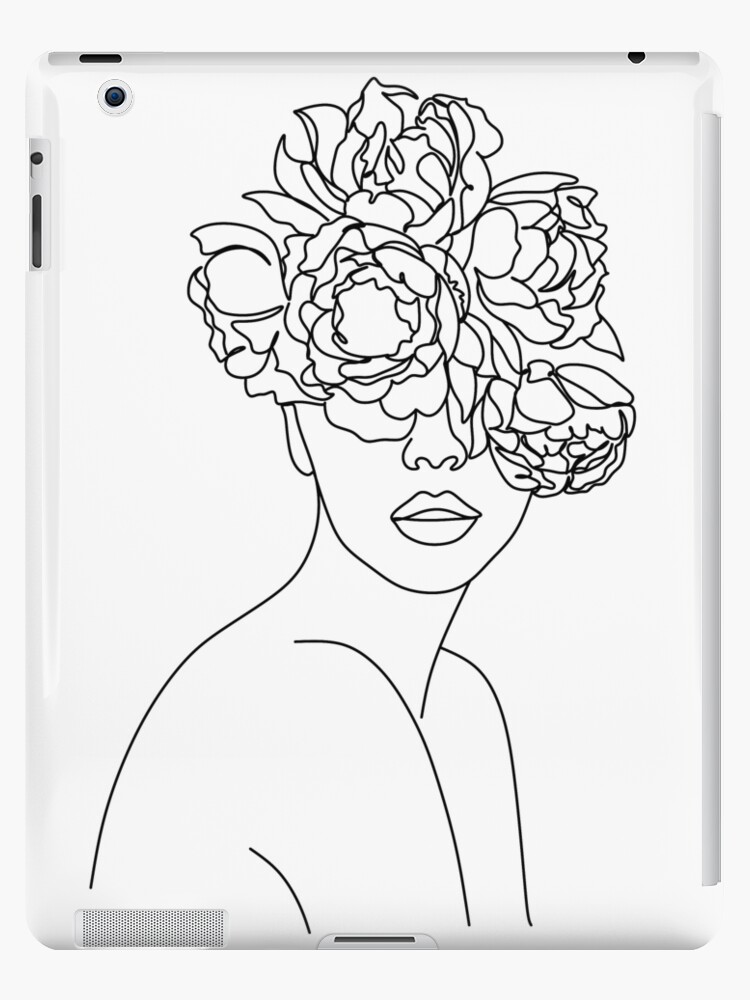This photograph features the back of a white or silver tablet, most likely an iPad indicated by the presence of traditional iPad buttons, including the volume, off button, headphone jack, and charging port at the bottom. The device also has a small black camera located at the top left corner and speaker holes at the bottom left. 

The tablet's back is embellished with a simple yet captivating line drawing of a woman, executed in plain black and white. The woman is depicted slightly hunched over, revealing her neck, arms, and the lower part of her face, which includes her nose and slightly open lips. Her right ear is also partially visible. Instead of the upper half of her face and head, the drawing transitions into an intricate bouquet of about five flowers, potentially roses or peonies, with abundant petals. These flowers obscure the top two-thirds of her face, extending from her forehead and substituting for her hair. The overall composition suggests that the flowers are emerging from her mind, creating a fusion of human and floral elements.